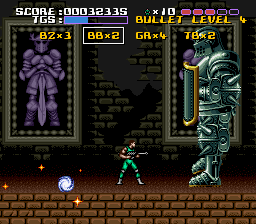In this colorful side-scroller video game screenshot, the scene features a detailed character and interface. The floor is constructed of brown bricks, and a small white swirl resembling a galaxy with some orange stars is visible on the left side of the image. The main character, dressed in green with green socks and white shoes, has muscular arms and short black hair. He holds a gray gun and faces the right, confronting a much larger medieval knight statue adorned in green armor with bronze accents at the feet, and a large green shield with gold detailing. This statue towers over the character at about five times his height.

The interface at the top of the screen shows various statistics: the score is displayed as "000,32335", beneath which the letters "TGS" appear. Adjacent to this, a blue bar, potentially representing health or energy, is filled to approximately one-third of its capacity. Below this are various counters: "BZ x3", "BB x2" (highlighted by a box), "GR x4", and "TB x2", accompanied by a bullet level indicator set to 4 and a vial icon labeled "x10". Additionally, there are five oval indicators, three of which are filled in pink.

In the background, the walls are a mix of olive green bricks and a darker green open section. Two large images of knights with large swords, outlined in olive green or mid-gray, frame the scene on both the left and right sides.